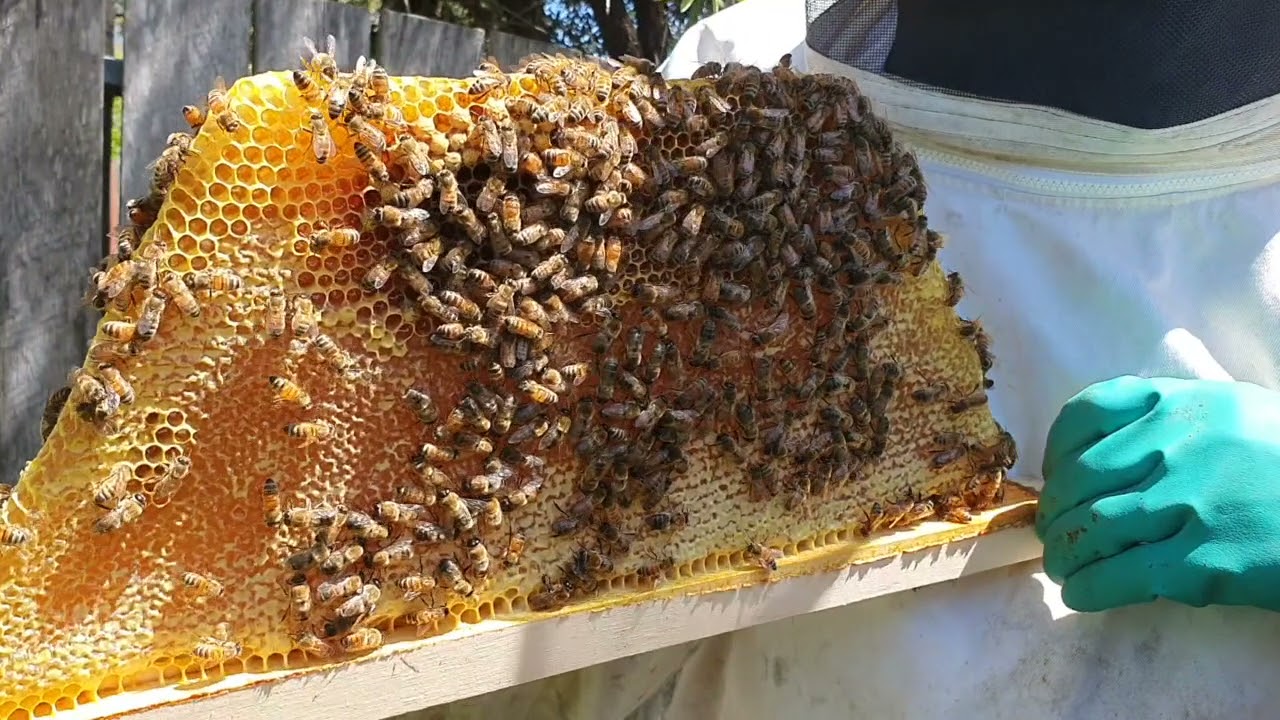The image captures a close-up of a large, cut-out piece of honeycomb from a beehive, teeming with an estimated 50 to 100 honeybees. The honeycomb, showcasing the classic hexagonal structure in varied sizes and textures, rests on a white wooden base. Portions of the comb appear filled with golden honey, particularly in the lower right, while the upper left is more vacant. The scene is set against a weathered, gray wooden fence, approximately five to six feet high, with a hint of a tree visible in the background. A beekeeper, identifiable by their white protective suit and black mesh facial covering, is holding the honeycomb with a turquoise-gloved hand, their torso prominently featured in the frame. The beekeeper carefully observes the bees as they crawl over the vibrant yellow-gold comb.